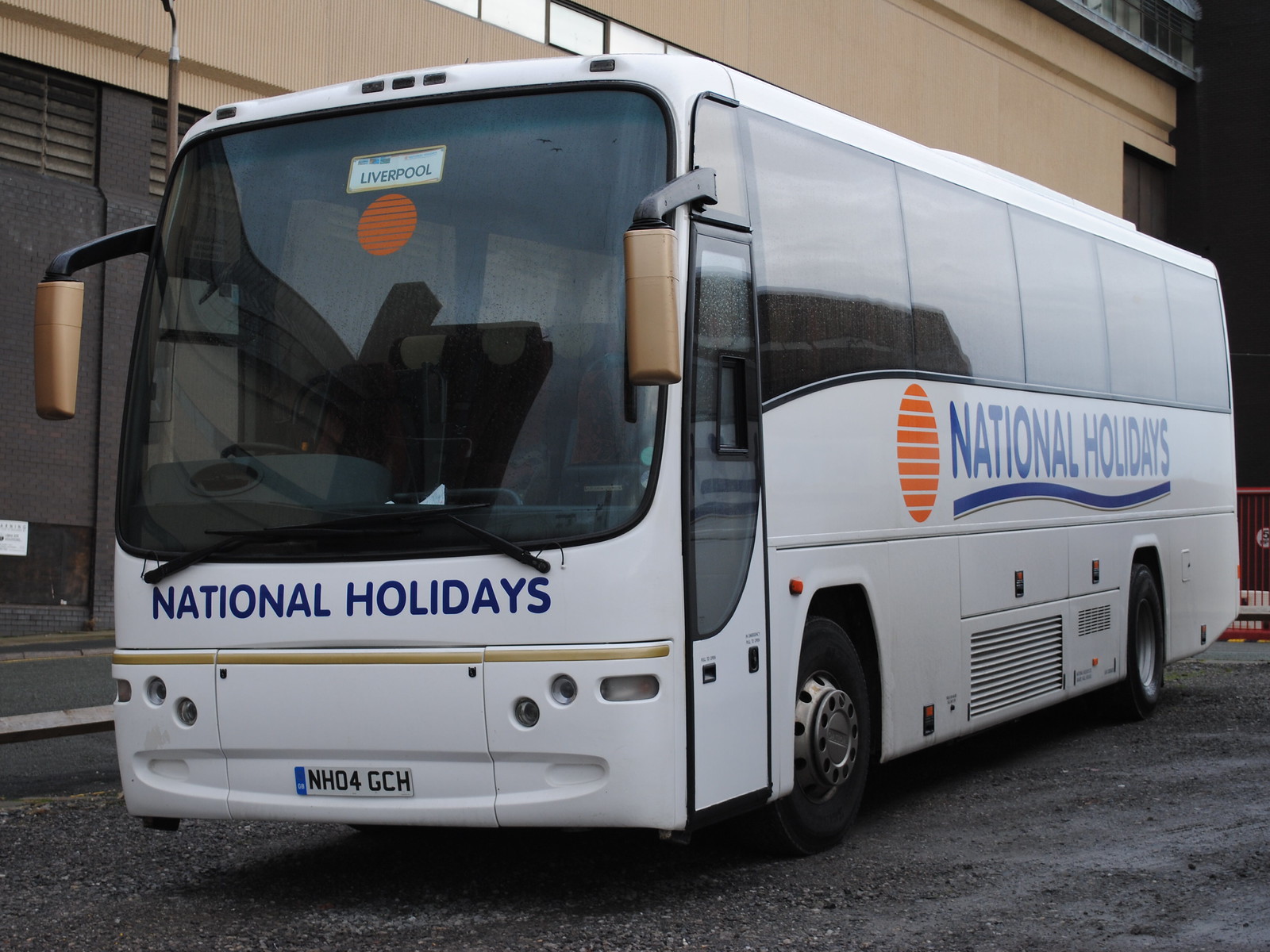The photograph captures a predominantly white bus, viewed from an angle that showcases both the front and the passenger side. The vehicle is branded with "National Holidays" in blue, prominently displayed on the hood and repeated along the side. Accompanying the text on the side is a distinctive logo: a curly blue line beneath the text and an orange circle with white horizontal lines cutting through it, matching the logo seen again below the destination label. The destination displayed through the front window reads "Liverpool" in black text on a white background. The bus features left and right side mirrors in a contrasting beige color. It is parked on a gravel road, with the background resembling a warehouse or large building. The license plate reads "NHD4GCH."